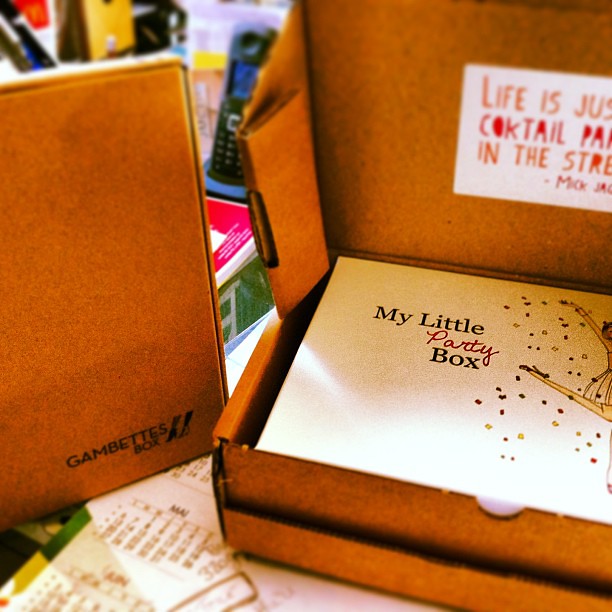The image depicts a cluttered indoor setting, potentially in a store, showcasing a variety of objects arranged on a desk. Dominating the right side of the image is an open brown cardboard box with a white sticker on the lid that reads, “Life is Just a Cocktail Party in the Streets,” followed by the name “Mick Jagger.” Inside this brown box, there is a white subscription-type box labeled "My Little Party Box," featuring an illustration of a woman in a dress celebrating amid confetti. Her pose is dynamic, standing on one leg with the other raised joyfully.

On the left side of the image, there is another cardboard box labeled “Gambit's Box.” Scattered around these boxes are additional items, including paperwork, a calendar or planner, a cordless phone, and some pens, adding to the overall sense of congestion. The scene is rich with colors such as brown, black, yellow, green, gray, orange, pink, and purple. The detailed arrangement and variety of objects suggest a lively, perhaps chaotic environment, likely within a store or a workspace.